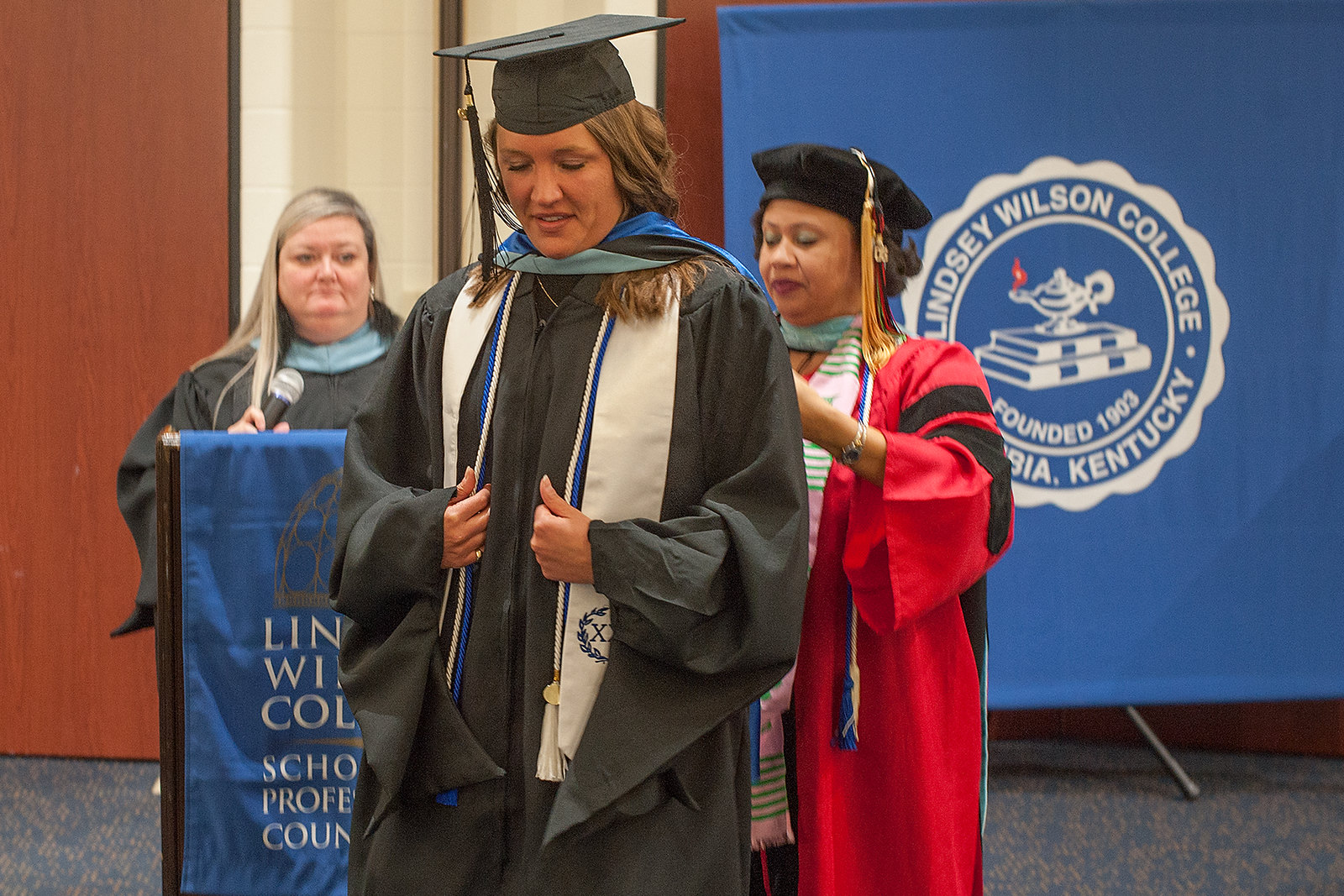The image depicts a graduation ceremony at Lindsay Wilson College in Kentucky. At the center, a young woman with long blonde hair is speaking into a black microphone with a silver tip, while standing at a podium adorned with a blue banner that reads "Lindsay Wilson College, Founded in 1903." She is dressed in a black jacket and black robe with a blue neckline.

To the side of the podium, a woman wearing a red cap with gold tassels, a red cape with black sleeves, and a black hat is assisting another young woman. This second young woman is wearing a black graduation gown and cap, and a white sash, signifying that she is about to receive an award or is being prepared for the next step in the ceremony.

In the background, there is another blue banner featuring the college's name and founding year, along with symbols of two books and a genie lamp. The scene captures the celebratory and formal atmosphere of the graduation event.